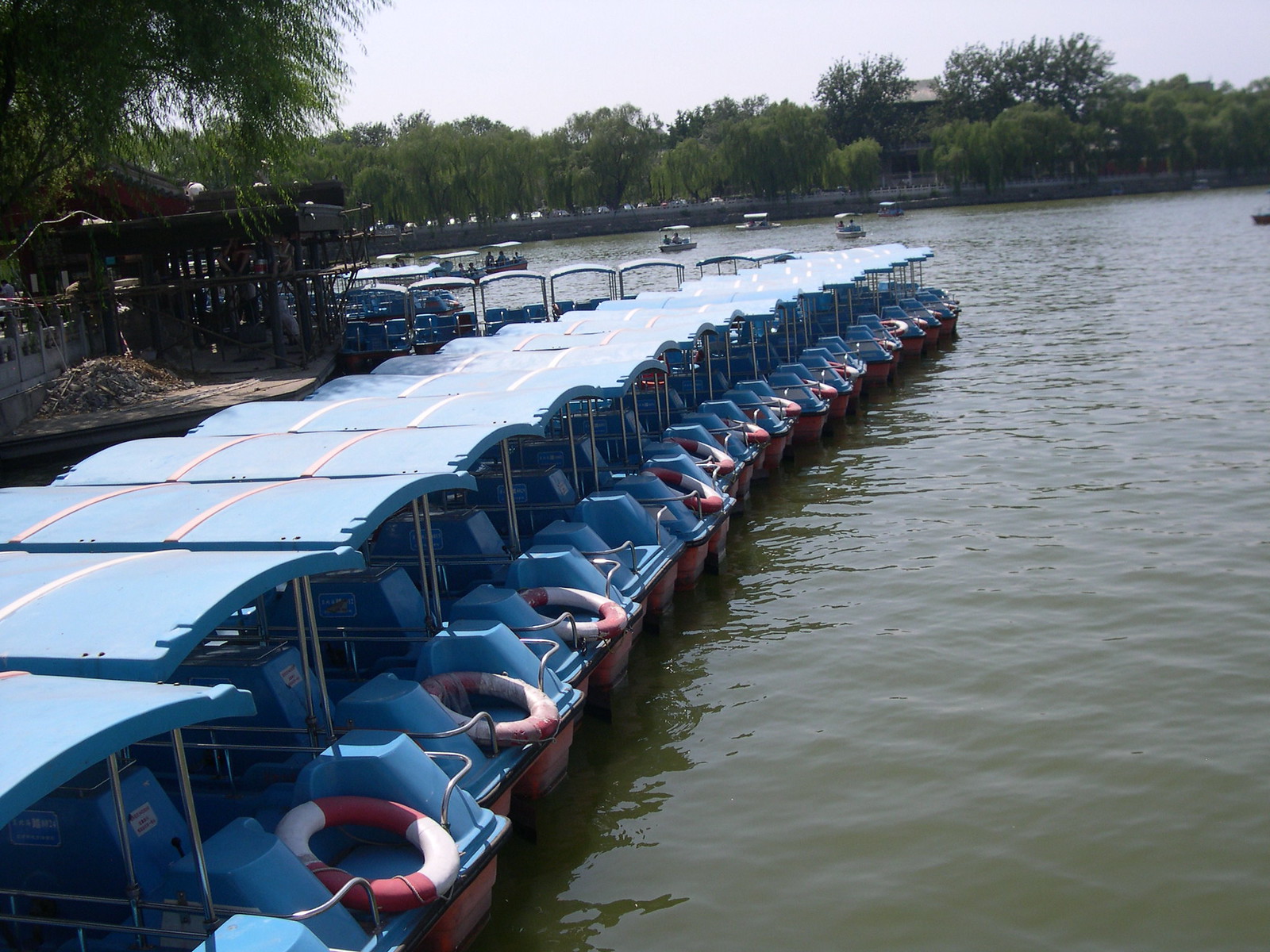The image depicts a serene lakeside scene with an array of paddle boats lined up along the shore. These boats, numbering about 15 to 20, feature blue canopies to shield from the sun and are equipped with red and white life-saving devices attached to their sterns. The lake water is a murky greenish-brown tone. On the left side of the image, there stands a wooden hut-like structure with a pile of branches nearby. In the distance, several paddle boats can be seen floating on the water, while the far shoreline is lined with lush green trees. In the backdrop, a barely visible house peeks through the dense foliage, adding a touch of human presence to the picturesque landscape.